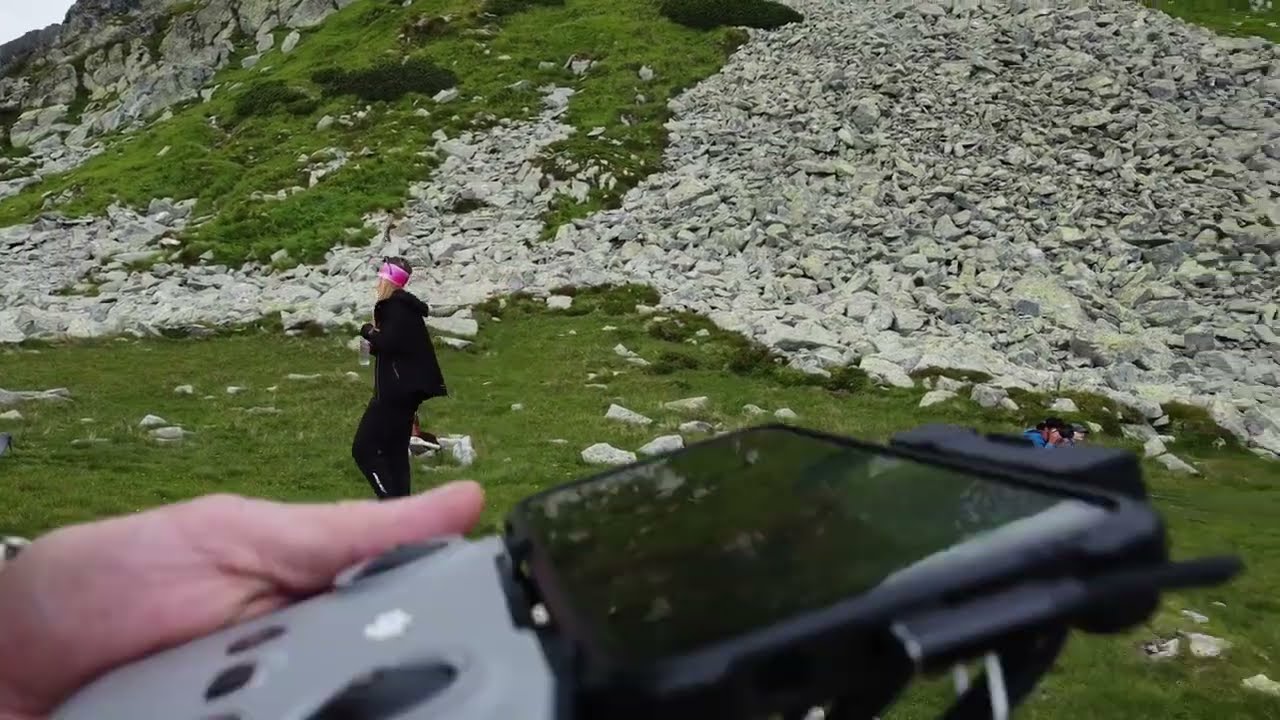The photograph, captured from a first-person perspective, prominently features a person holding a gray and black drone controller in the foreground, their hand slightly out of focus. The controller has a view screen on top, hinting at a possible connection to a smartphone or other device, and dominates the bottom portion of the image. Beyond this, the scene unfolds to reveal a grassy field interspersed with patches of white-gray rocks. To the left, there is a man dressed in a black outfit with a distinctive red headband, walking away from the viewer. Behind him, the landscape slopes upward with a mix of grass and rock, culminating in a towering, partially visible cliff of solid rock towards the upper left. In the upper right corner, another man appears to be crouching, possibly holding a camera. The photograph includes a mix of colors, including black, white, gray, brown, green, pink, and peach, and captures the scene in a realistic and unpolished manner, suggesting it was taken spontaneously rather than professionally.